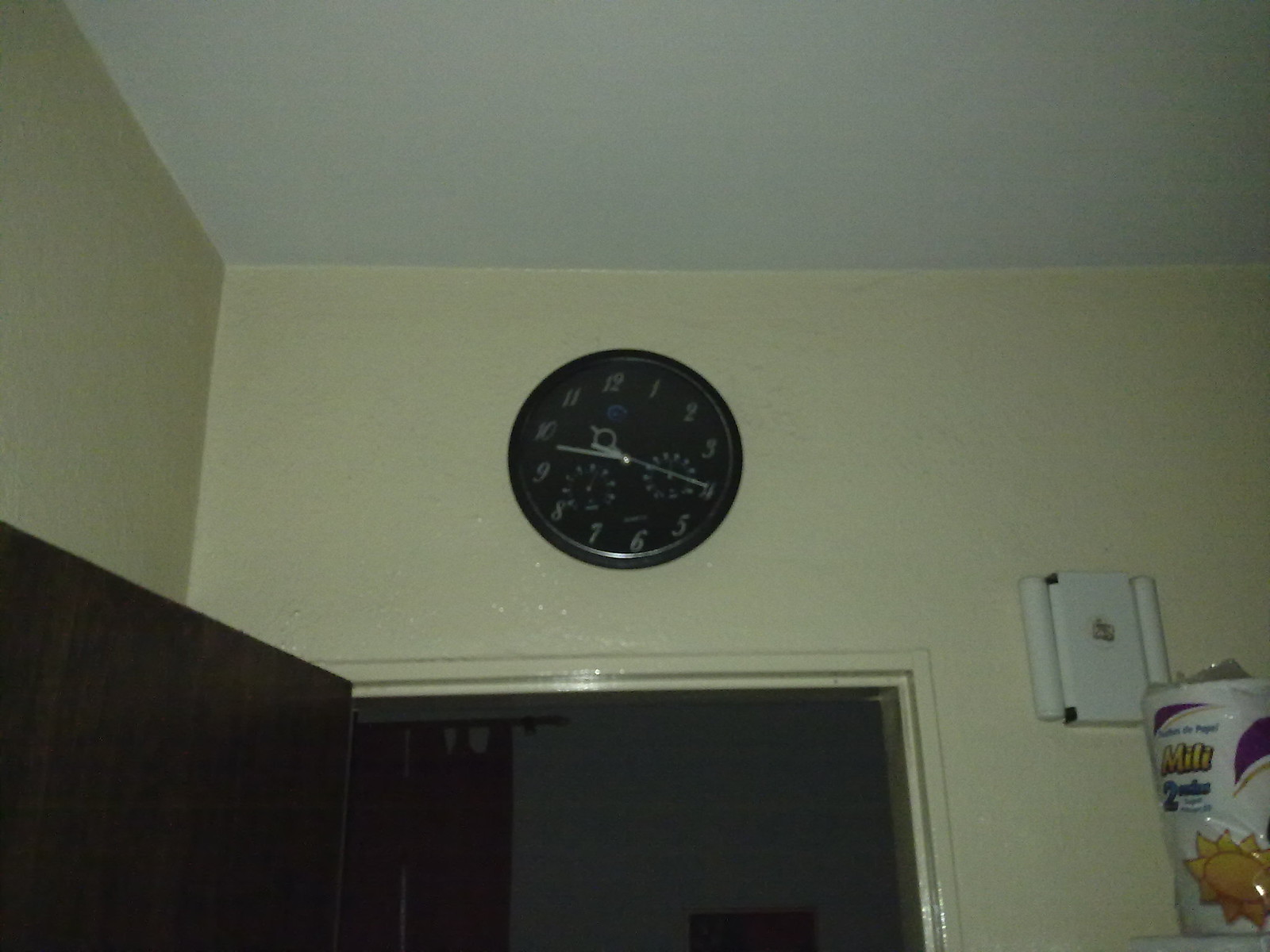This photograph captures the inside of a room, providing a detailed view above a doorway. Dominating the wall above the doorway is a black circular clock with white numbers and hands, currently showing a time between 9:30 and 10:00. 

In the lower left-hand corner, the door frame is visible, showing a darker room beyond with a door that appears to be either dark brown or nearly black. This darker room contrasts sharply with the well-lit area in the foreground. 

On the lower right-hand side of the image, there is a white package with a yellow drawing of a sun resting against the wall. Above this package, a white rectangle, likely a switch or control panel, is mounted on the wall.

The detailed elements, such as the contrasting colors and specific positions of objects, create a rich visual narrative of the space depicted.